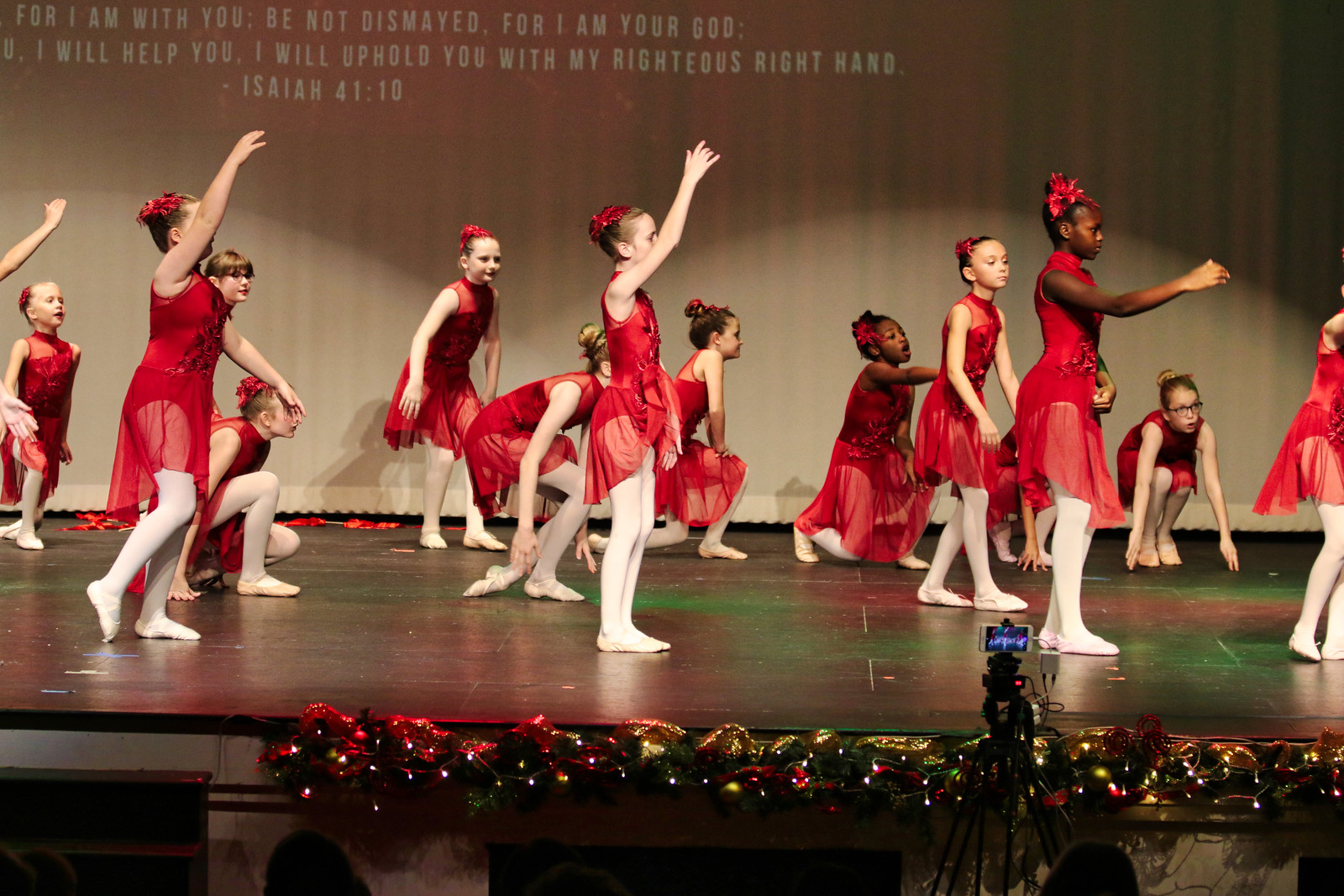The photograph captures a diverse group of young girls performing on a stage, all dressed in sleeveless red ballet dresses with see-through bottoms that reveal red underwear, complemented by white stockings and ballet slippers. Each girl has her hair styled in a bun adorned with a red or yellow bow. They are engaged in a ballet performance with various poses: some have their hands raised, others are squatting, and some have their arms stretched out. The scene suggests Christmastime, evidenced by the Christmas decorations lining the front of the stage. A tripod-mounted camera is also visible, recording their performance. In the background, a project text from Isaiah 41:10 reads, "For I am with you; be not dismayed, for I am your God; I will help you, I will uphold you with my righteous right hand."